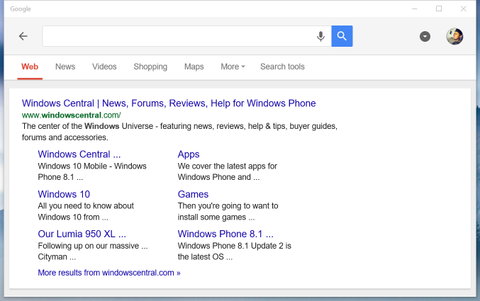Screenshot of a Google search results page with a white background. At the top, "Google" is displayed in gray text, accompanied by a search bar featuring a blue magnifying glass icon. Below the search bar is a navigation bar with various tabs: "Web," "News," "Videos," "Shopping," "Maps," "Store," and "Search tools." The "Web" option is highlighted in red. 

Below the navigation bar, a blue text link reads "Windows Central - News, Forums, Reviews, Help for Windows Phone," followed by a green URL, "www.windowscentral.com." Beneath that, in black text, is a description: "The center of the Windows universe, featuring news, reviews, help and tips, buyer guides, forums, and accessories."

Further down, two columns of options are presented. The first column includes links related to "Windows Central," "Windows 10 Mobile," "Windows Phone 8.1," and "Windows 10," with subtext like "all you need to know about Windows 10 from our Lumia 950XL," and references to a "massive city man." The second column covers "Apps," mentioning "the latest apps for Windows Phone and games," and "Windows Phone 8.1," detailing that "Windows Phone 8.1 Update 2 is the latest OS." At the very bottom, a blue link indicates "more results from windowscentral.com."